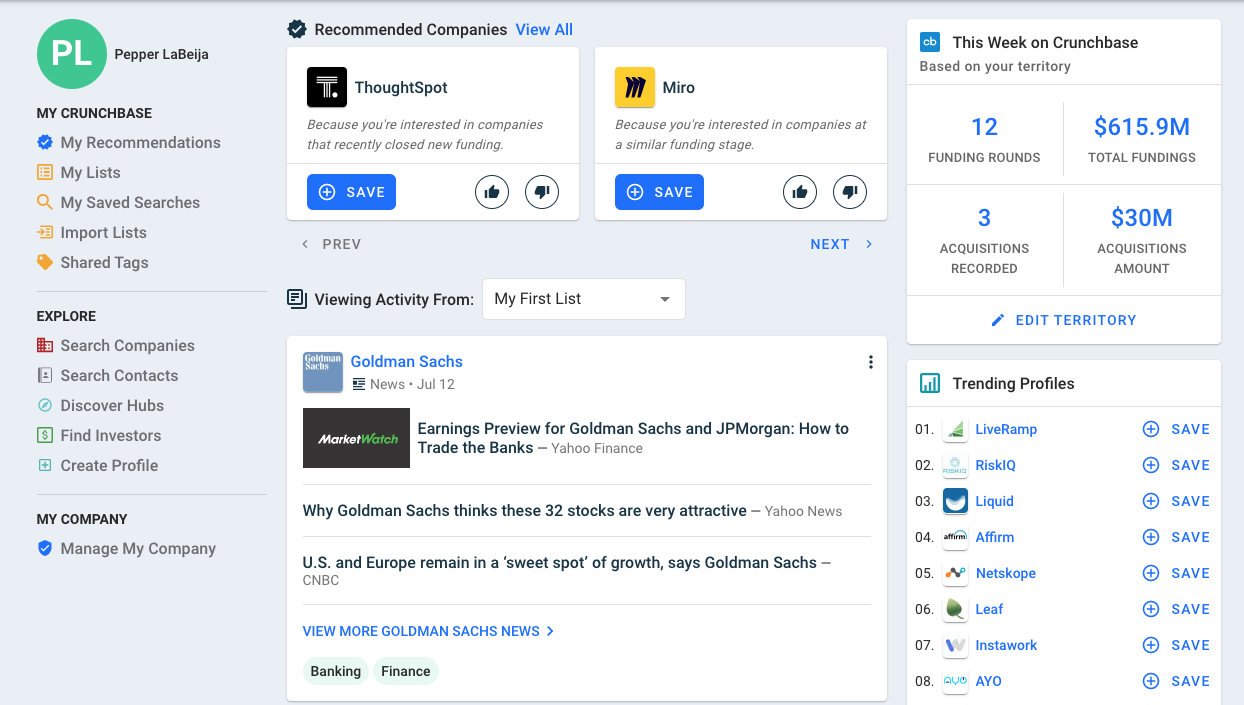Screenshot of the Crunchbase Dashboard:

In this detailed view of the Crunchbase user interface, we observe several key elements. At the top-right corner, there is a white "CB" logo set against a blue background, indicating the Crunchbase branding. Adjacent to this logo, a heading reads "This Week on Crunchbase," followed by the subheading "Based on Your Territory". 

Below this section, there are two rows, each divided into categories. The first category reports "12 Funding Rounds" with a combined total of $6.159 million in funds raised. Additionally, it lists "3 Acquisitions Recorded" amounting to $30 million. A button below these statistics allows users to edit the displayed information. 

Further down, links to various trending profiles are visible, hinting at its stock-related nature, though not confirmed. On the top-left corner, the logged-in user's name, "Pepper LaBija," is displayed, with several personalized navigation links underneath: "My Recommendations," "My List," "My Saved Searches," "Important Listings," and "Shared Tags". 

Below this section, options for exploring different companies and managing them are provided, with relevant links positioned at the bottom left. Central to the interface, recommended companies are listed, and beneath them, there is a feature to search viewing activity within a specified time range.